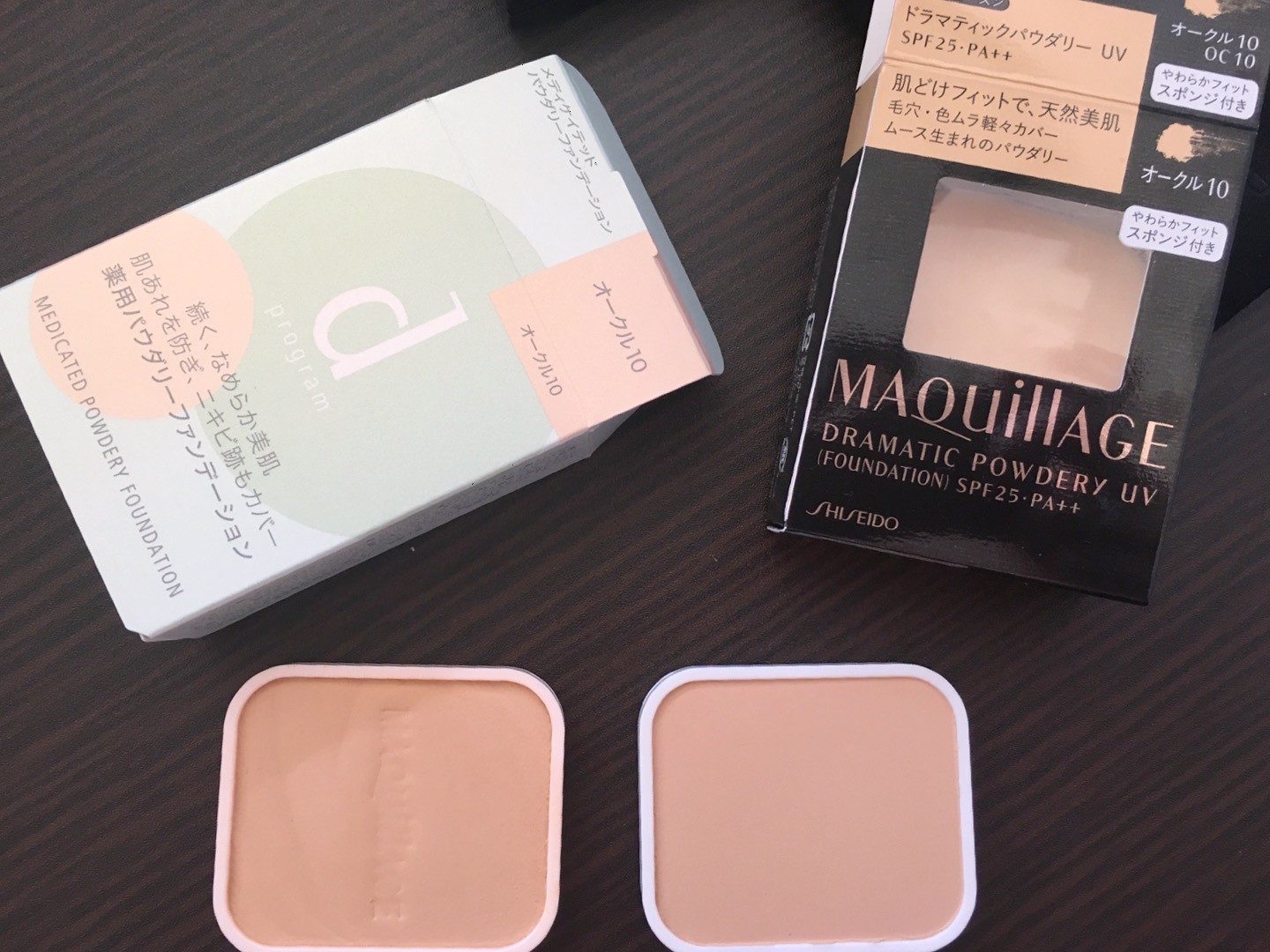The image depicts a close-up shot of two distinct makeup products placed on a dark wood tabletop. These items appear to be of Asian origin, likely from Japan or South Korea, as suggested by the packaging design and language. 

On the left side, there is a package for the "Malolage Dramatic Powdery UV Foundation SPF 25 PA." The packaging is primarily black with a combination of tan and white text. Below this box lies the container of the foundation itself.

On the right side, another packaging features a pastel color scheme with shades of tan, green, and blue. At the center of the package, a pastel green circle encloses the letter "D". The legible English text on this packaging reads "Medicated Powdery Foundation." Similar to the first product, its respective foundation container is positioned beneath the box.

Both products are meticulously arranged, highlighting their distinct packaging and containers, which sit side by side on the elegant wooden surface, enhancing the aesthetic appeal of the composition.